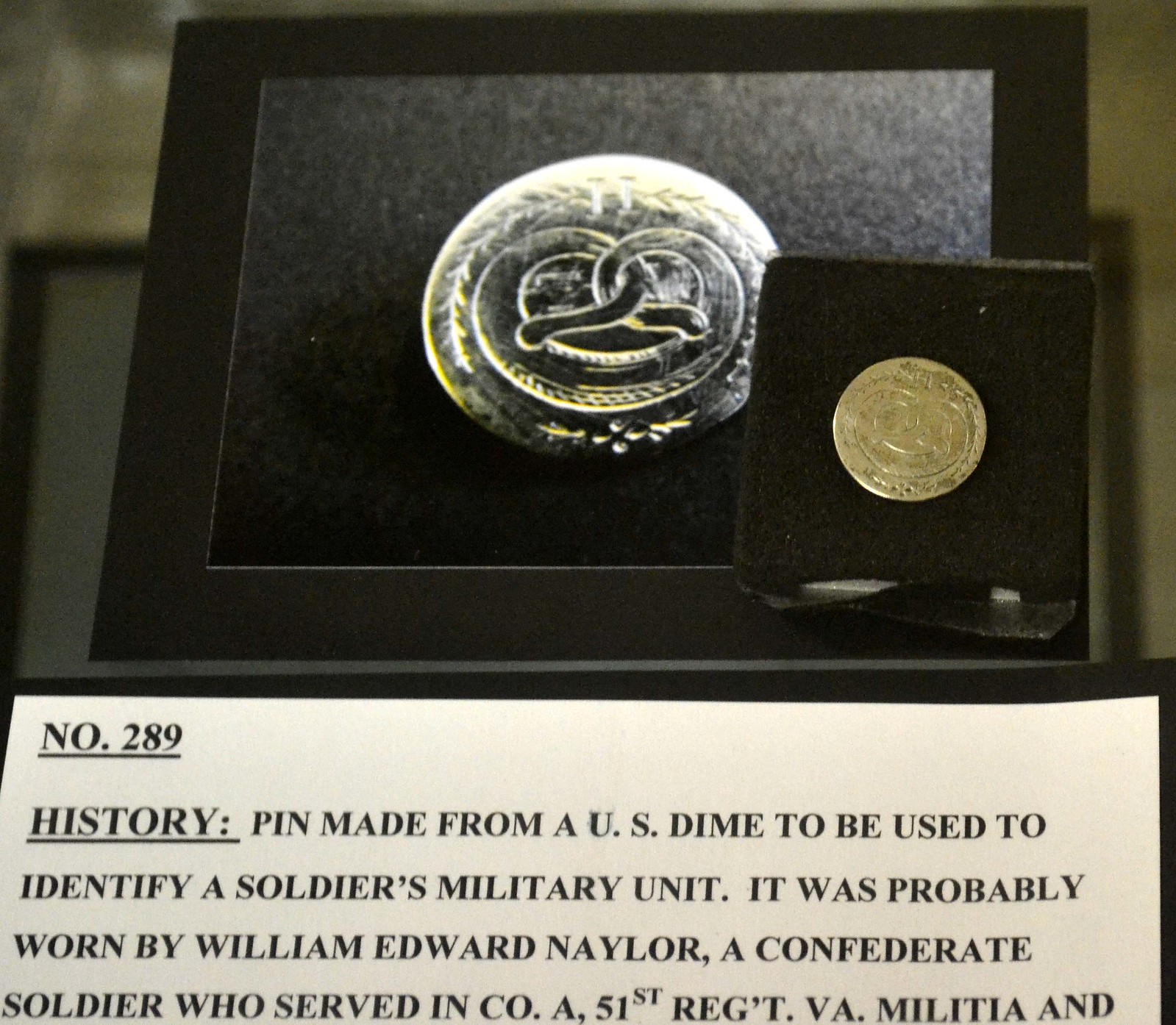This close-up image captures a detailed museum display centered around a historical pin, made from a U.S. dime, used to identify a soldier's military unit. The display showcases two representations of the pin against a black background: a significantly worn and faded silver pin positioned on a piece of black felt, and a larger, more detailed photograph of the same pin framed behind it. The image highlights matching elements between the physical pin and its photographic representation, emphasizing the intricate engravings. Below these items, a sign numbered 289 provides historical context, stating that the pin was likely worn by Confederate soldier William Edward Naylor, who served in Company A of the 51st Regiment, Virginia Militia. The sign's remaining text is cut off, with the visible portion written in black type on a white background.